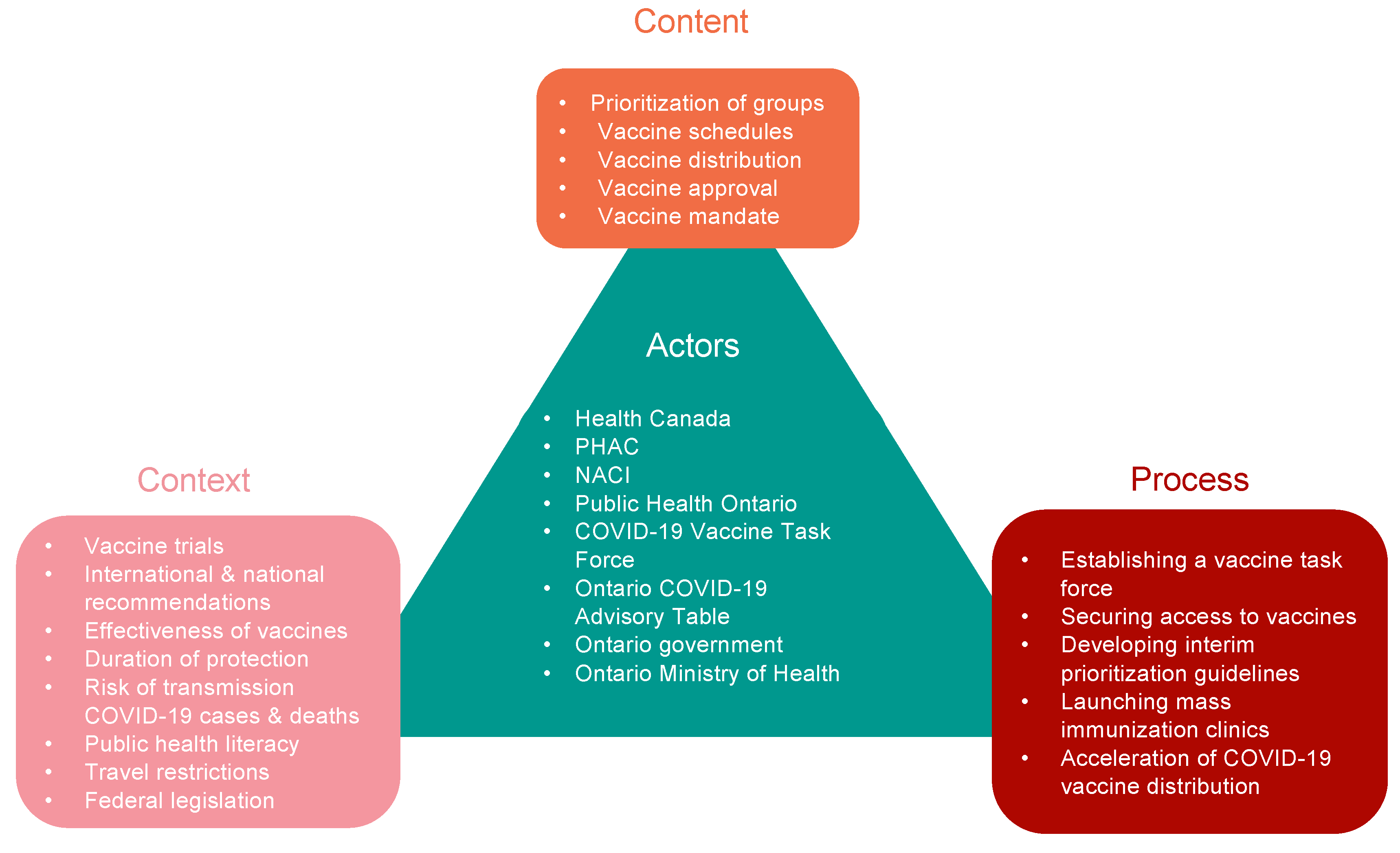This diagram is a detailed flowchart depicting various aspects of vaccine management, represented by different shapes and colors. At the center is a turquoise triangle labeled "Actors," listing entities such as Health Canada, PHAC, NACI, Public Health Ontario, COVID-19 Vaccine Task Force, Ontario COVID-19 Advisory Table, Ontario Government, and Ontario Ministry of Health. Surrounding this central triangle are three rounded squares, each connected to a vertex of the triangle.

At the top vertex, an orange rounded square labeled "Content" outlines critical points like the prioritization of groups, vaccine schedules, vaccine distribution, vaccine approval, and vaccine mandates. The bottom left vertex features a pink rounded square labeled "Context," which details considerations such as vaccine trials, international and national recommendations, effectiveness of vaccines, duration of protection, risk of transmission, COVID-19 cases and deaths, public health literacy, travel restrictions, and federal legislation. Finally, the bottom right vertex presents a red rounded square labeled "Process," highlighting steps such as establishing a vaccine task force, securing access to vaccines, developing interim prioritization guidelines, launching mass immunization clinics, and accelerating COVID-19 vaccine distribution.

Each section of the diagram is meticulously itemized with white bullet points, ensuring a clear and comprehensive depiction of the multi-faceted approach to vaccine management.